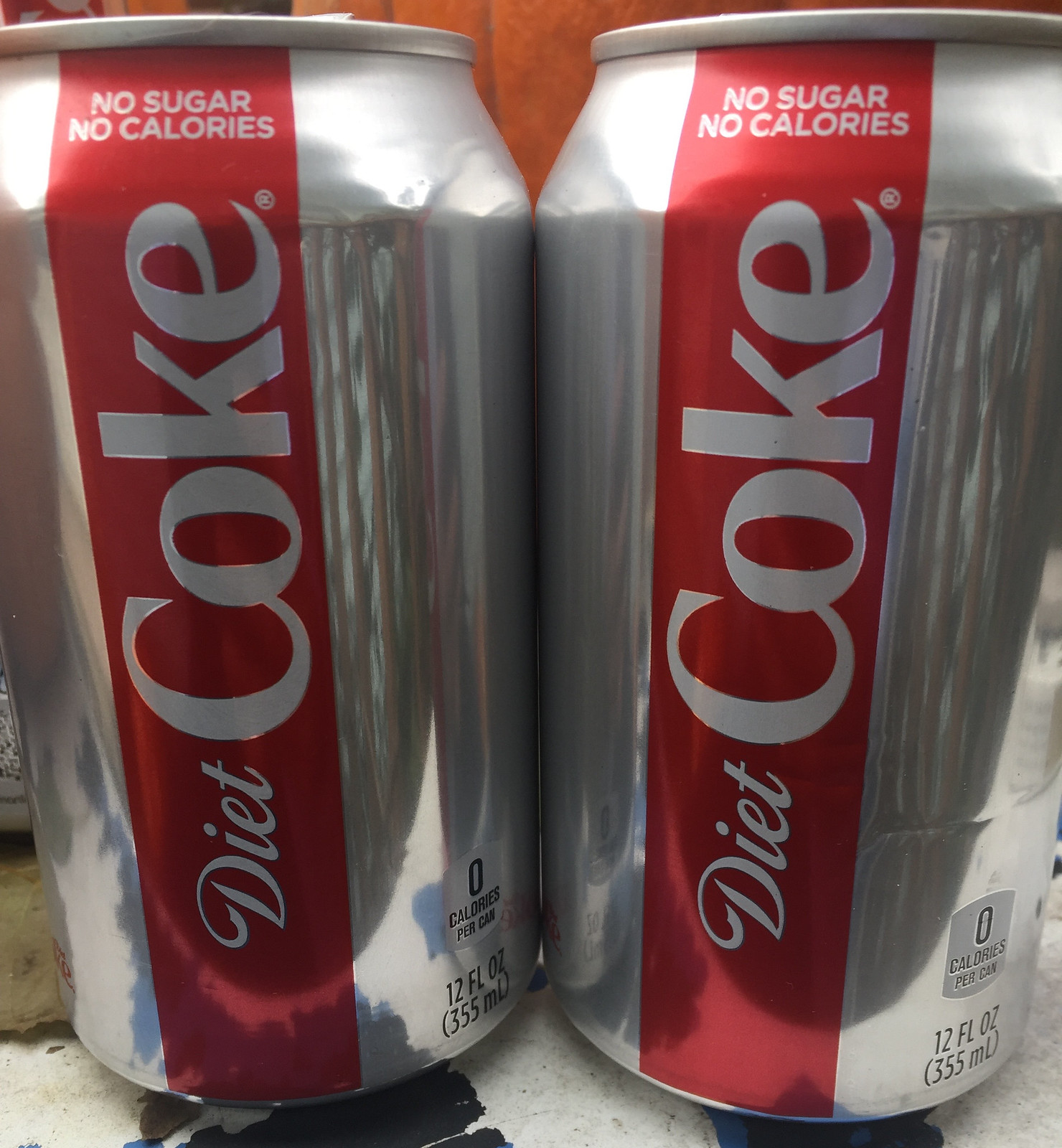The image features two silver aluminum Diet Coke cans prominently displayed on a contrasting surface. The surface seems to be a combination of black ink, forming an abstract blotch, overlaid on white paper with hints of brown undertones peeking through. Each can is adorned with a bold red vertical streak running down the center and showcases the white text "Diet Coke," and the phrases "no sugar" and "no calories." A distinctive black zero in a gray box indicates the calorie content, and the volume of the cans is clearly marked as 12 fluid ounces or 355 milliliters. The vivid red wall in the background adds a striking pop of color that complements the red accents on the cans, creating a visually engaging contrast against the monochromatic tones of the foreground.